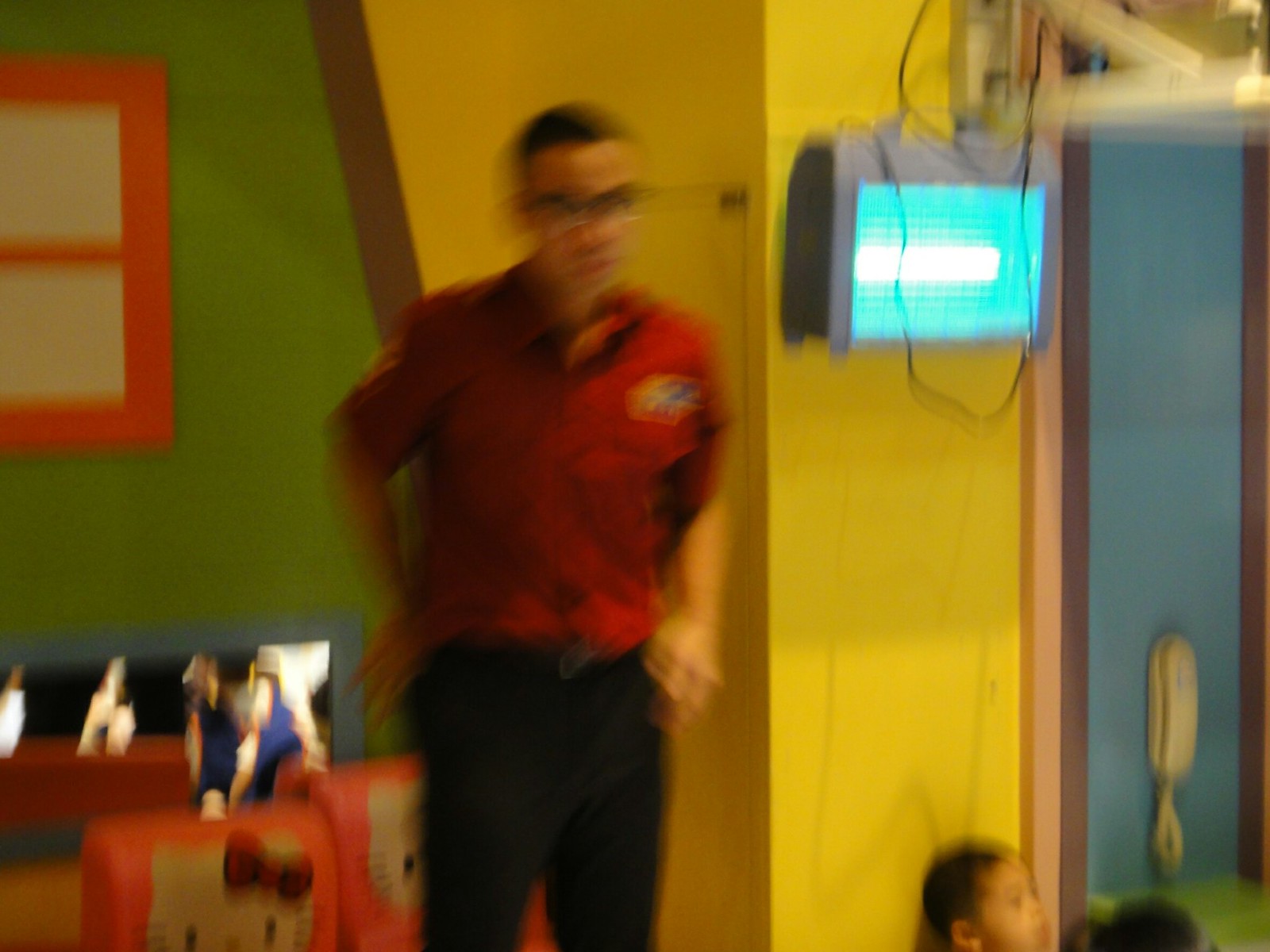A person in a uniform, wearing glasses and a red shirt adorned with a name tag, stands centrally in black pants. Behind them, a large screen is visible, set against vibrant and multicolored walls. The backdrop features a yellow wall merging into a green section with an orange board, filled with white cards. Adding to the playful atmosphere, a mirror decorated with Hello Kitty motifs catches the eye. An older model white phone is positioned nearby, suggesting the image could be from an earlier time. In one corner, several children are gathered, hinting that the setting might be a daycare or a festive venue for children's birthday parties. The overall environment, with its colorful walls and whimsical decoration, exudes a cheerful space designed for kids' activities and celebrations.